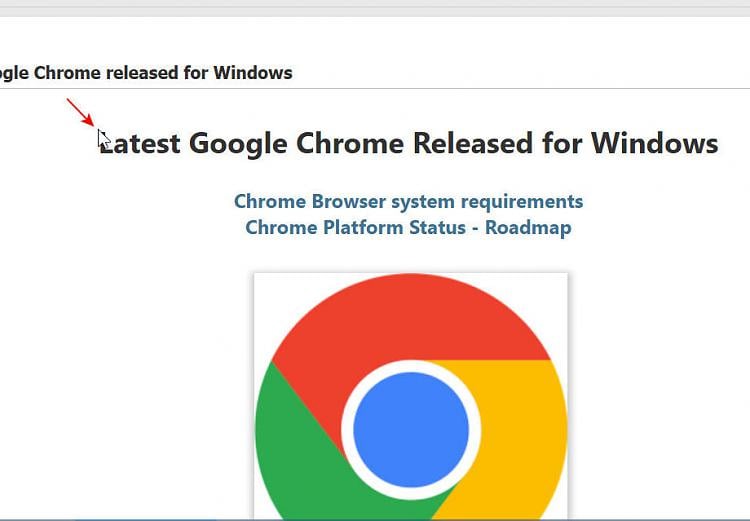The image is a screen capture of an infographic with a white background. At the top, black text reads "Google Chrome Released for Windows." Directly beneath this, the text continues with "Latest Google Chrome Released for Windows." A thin, red arrow is pointing towards the "L" in "Latest," and a white mouse cursor is also visible over this "L." Below this, you see blue text that states "Chrome Browser System Requirements" and "Chrome Platform Status - Road Map."

Central to the image is a large, round Google Chrome logo, showcasing its distinct colors: green, red, gold, with a blue dot at the center surrounded by white. The image has a thin gray bar at the top, and another thin gray line below the Google Chrome logo. The detailed area around the logo appears slightly pixelated, enhancing the visual emphasis on the logo. The rest of the image remains clear with no additional notable features.